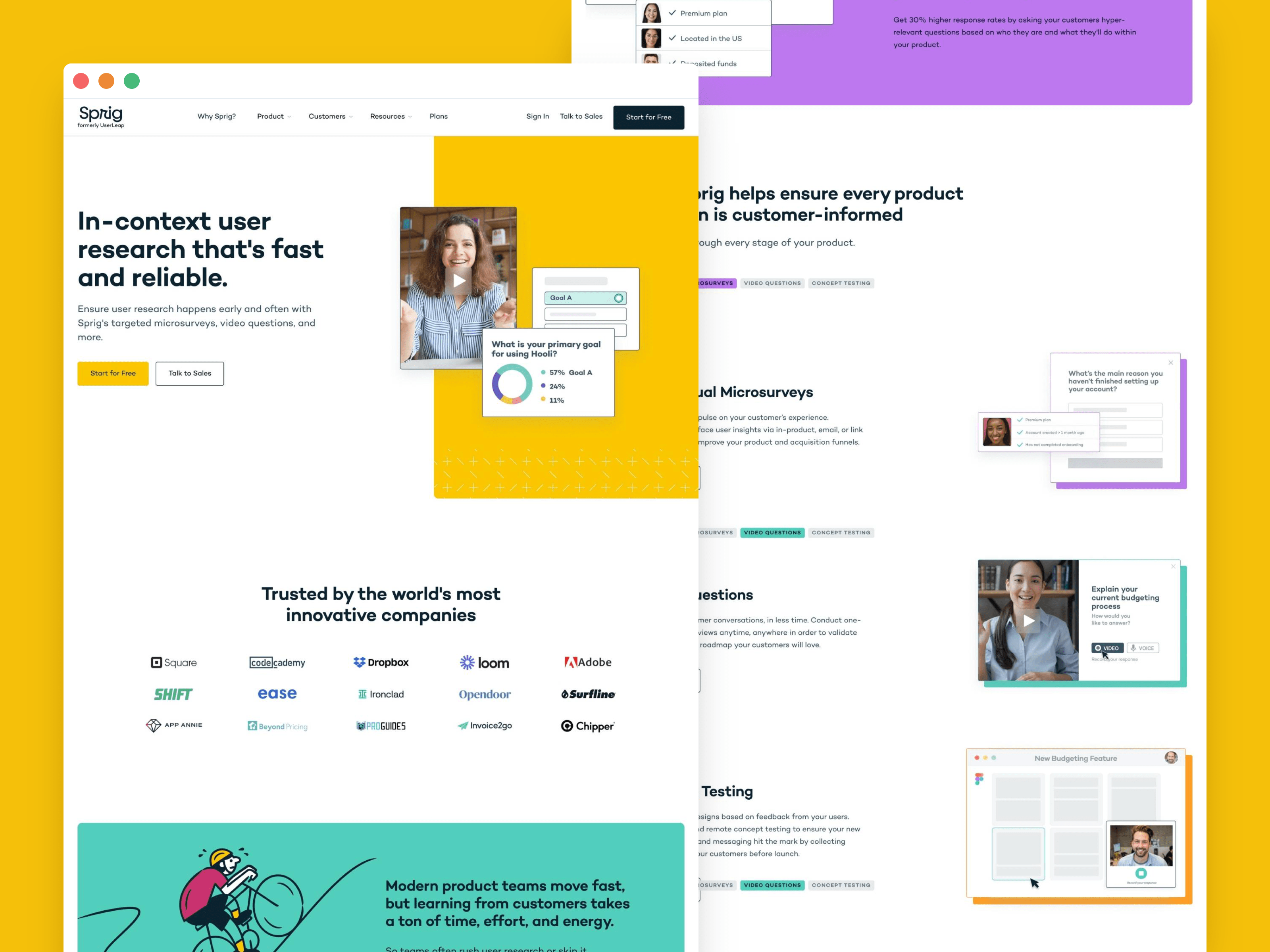Here is a cleaned-up and detailed caption for the image:

---

The image features a screenshot of a web page, presumably from a service called SPRDG, displayed prominently in the upper left corner. The SPRDG web page is layered on top of another web page, both set against a mustard yellow background. 

The top, smaller web page features the SPRDG logo at its upper section, characterized by three colored dots (red, orange, and green) reminiscent of the buttons on a browser window. The main header on this page, written in bold black text on a white background, states: "In-context user research that's fast and reliable." 

Beneath this header, there's a block of smaller black text that reads: "Ensure user research happens early and often with SPRDG's large [something], surveys, video questions, and more." However, part of this text is obscured or too tiny to decipher clearly.

The page also includes a prominent call-to-action in the form of two buttons. The first button is orange-yellow with the text "Start for free," while the second button is white with text that is unreadable due to its small size.

To the right side of the page, there is a video thumbnail featuring a smiling woman with long brown hair, dressed in a pinstripe blouse. This thumbnail includes a video play button and is accompanied by two white boxes, whose text content is too small to be legible.

At the bottom of this inset page, against a white background with black text, is a tagline reading: "Trusted by the world's most innovative companies," followed by a list of 15 companies' logos.

The larger web page visible behind this prominently displayed one seems to contain additional information, though the details are less clear.

---

This caption offers a comprehensive and clear description of the image, capturing all notable elements and their relative positions.